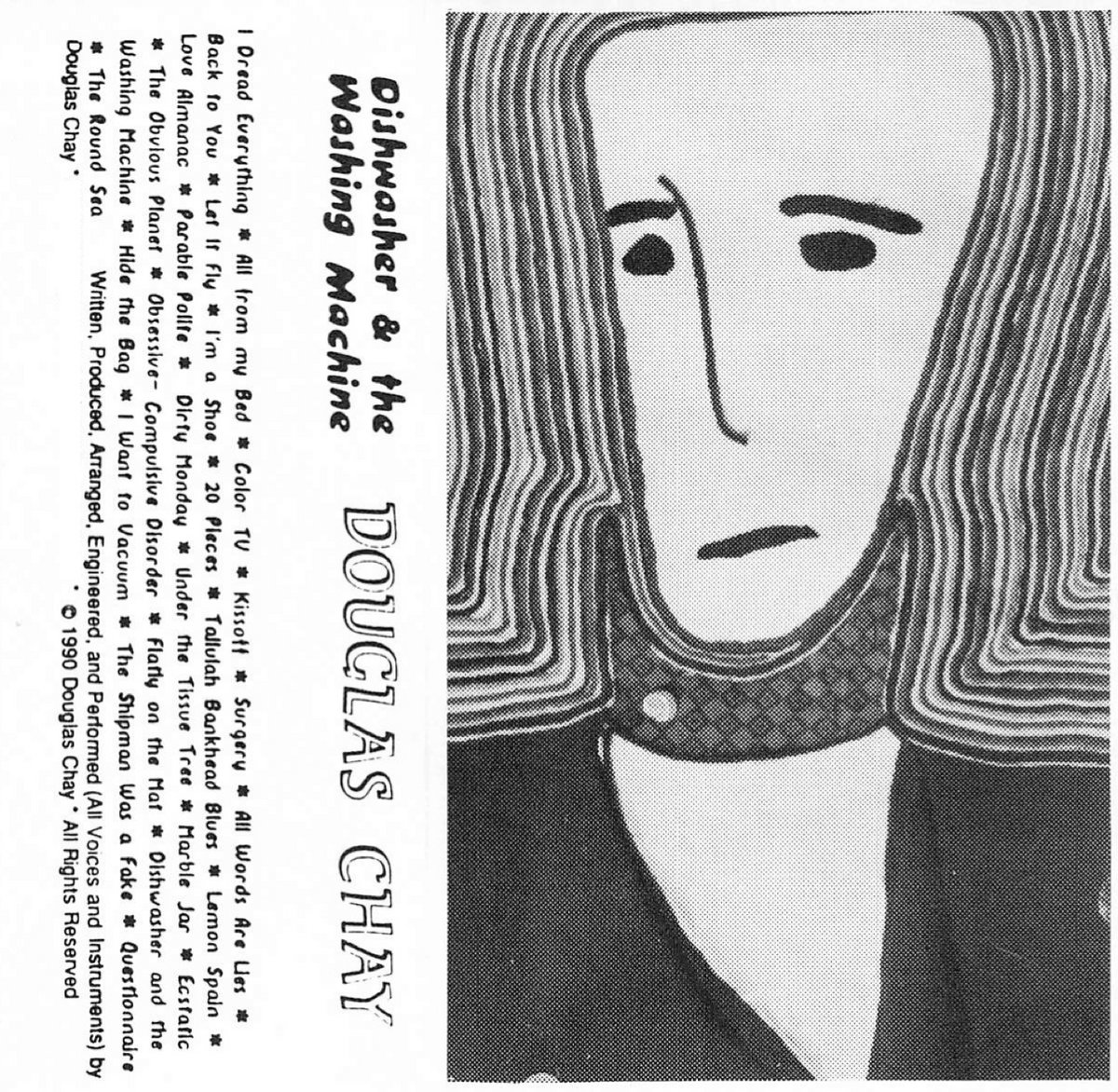The image appears to be the back cover of an album by Douglas Che, entitled "Dishwasher and the Washing Machine," featuring a black and white color scheme. On the left side, vertically oriented text lists various phrases and song titles, such as "I dread everything," "color TV," and "kiss off surgery." Other notable texts include "all words are lies," "obsessive compulsive disorder," and "flatly on the mat." At the bottom, it mentions all songs were written, produced, arranged, engineered, and performed by Douglas Che, with a copyright date of 1990.

On the right side of the image, there is a colorful, abstract drawing that resembles a child's depiction of a person. The figure has a candy corn-shaped head with minimal facial features and is dressed in a black shirt and scarf. The drawing includes vibrant marker lines that radiate around the head and shoulders, giving it a halo-like effect. The figure appears to convey a worried or scared expression. Surrounding the image are scattered textual elements, adding to the album's eclectic and introspective vibe.